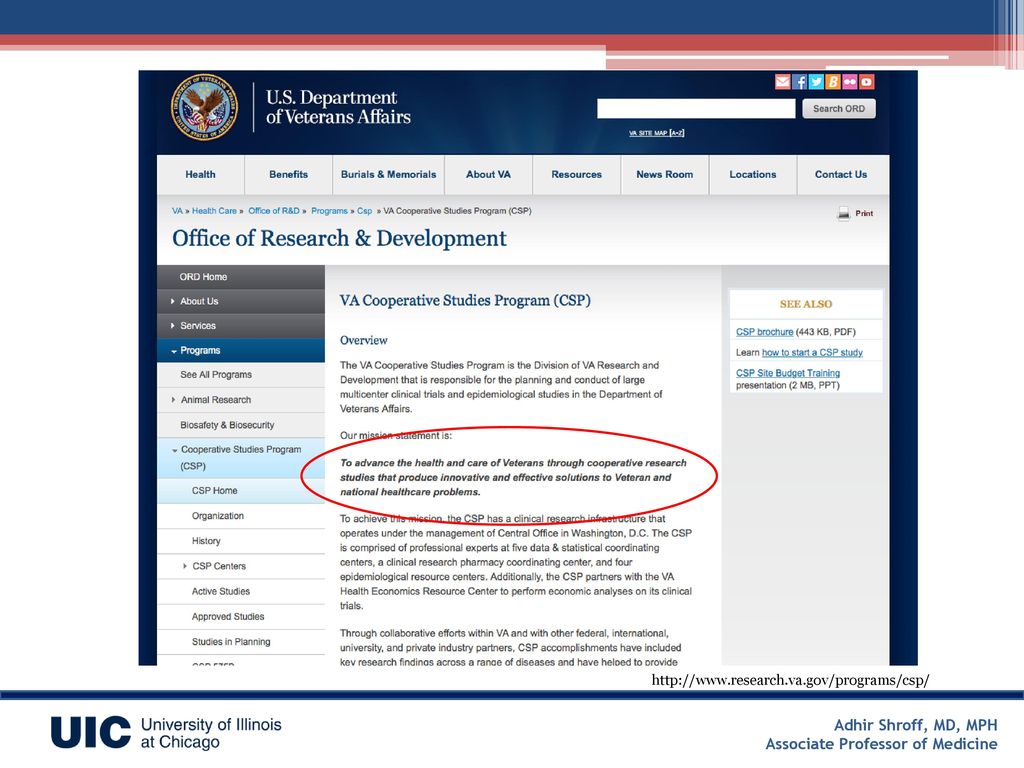This image is a landscape-oriented screenshot featuring various elements related to veteran healthcare research. 

At the center, a red circle highlights a prominent statement in bold and italics: **_To advance the health and care of veterans through cooperative research studies that produce innovative and effective solutions to veteran and national health care problems._** 

In the bottom left-hand corner, the University of Illinois at Chicago (UIC) logo is visible. Adjacent to it, in the bottom right-hand corner, there is text reading "ADHIR Shroff MD MPH, Associate Professor of Medicine," with a blue stripe above this information. To the right of that, the URL "www.research.va.gov/program/CSP" is displayed.

The upper section of the image features a gradient stripe transitioning from blue to red to pink, spanning from the left to the right corner. Positioned here is the US Department of Veterans Affairs logo.

Across the top portion, a series of menu options are listed: "Health Benefits, Burials and Memorials, About VA, Resources, Newsroom, Locations, Contact Us." Below this, the heading "Office of Research and Development" is displayed.

The main content is organized into three columns discussing the VA Cooperative Studies Program (CSP) — a division of VA Research. The narrative emphasizes the program's significance, mentioning its collaboration with colleges to interview veterans and address their needs.

Overall, the screenshot captures a detailed overview of collaborative efforts in veteran healthcare research, guided by the VA Cooperative Studies Program.